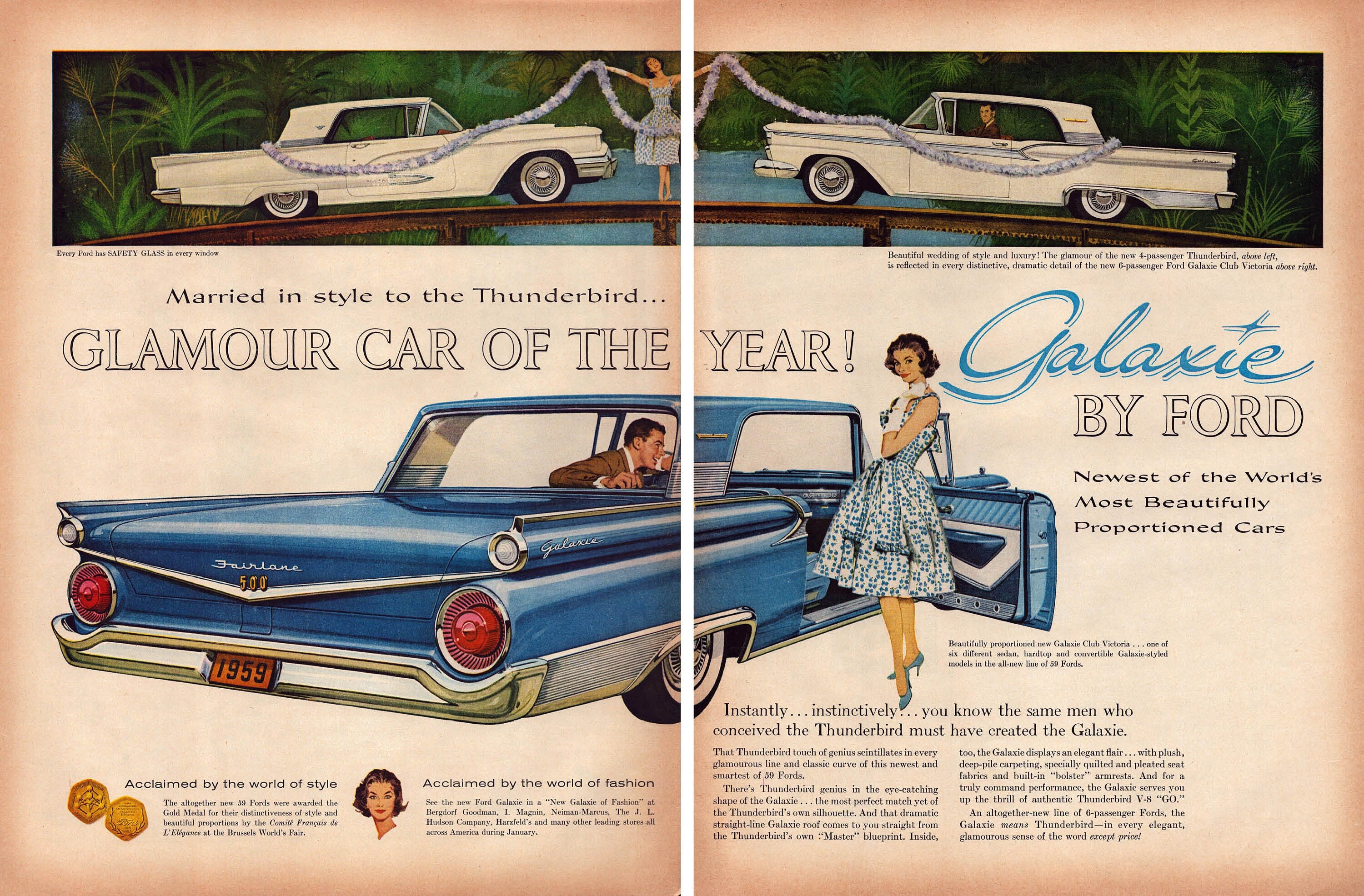The image is an old advertisement for the "Glamour Car of the Year," featuring the Galaxy by Ford. It showcases a vintage, blue car with a man in a brown coat sitting in the driver's seat, gazing at a woman standing by the open passenger-side door. The woman is dressed in retro 1950s attire, including a blue knee-length dress, blue pumps, and a classic curly bob hairstyle. The caption "Galaxy by Ford: Newest of the world's most beautifully proportioned cars" is prominently displayed. The ad also includes a detailed illustration in the upper section, showing two white vintage cars facing each other on a wooden bridge over a river with trees in the background. The same woman is seen standing between the cars, adding to the sense of glamour and sophistication. The bottom of the image contains a few paragraphs of text that are too small to read clearly, highlighting the car's features. The overall layout mimics an open magazine spread, split down the middle, giving it a distinctive 1950s vintage aesthetic.